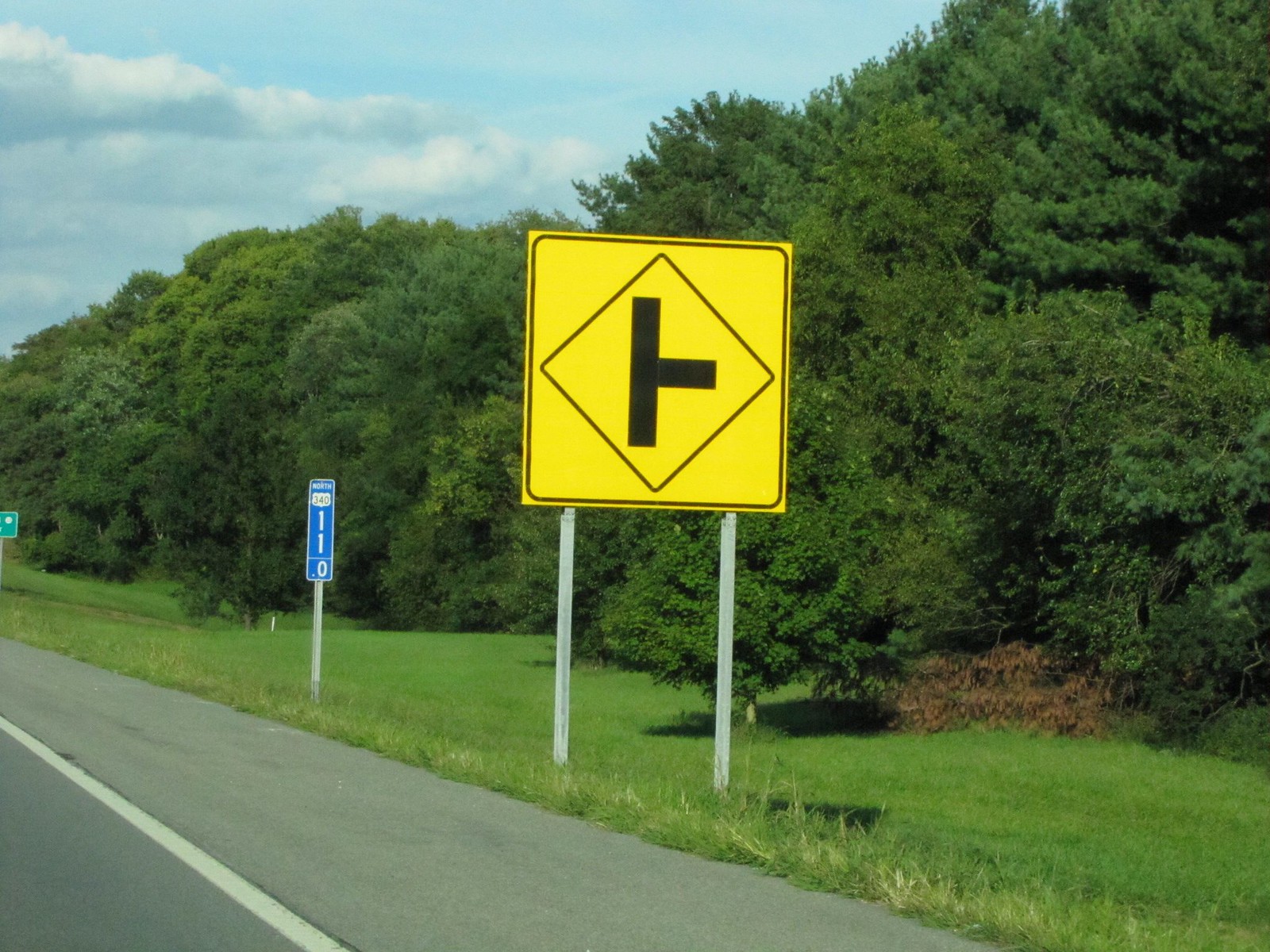The image captures a road situated in the left-hand corner of the frame, featuring two lanes separated by a distinct white solid line. Adjacent to the road is a grassy verge that gently slopes downwards, leading to a dense cluster of trees. The sky overhead is predominantly blue, interspersed with greyish-bluish clouds, giving it a somewhat overcast appearance. 

On the right side of the image stands a prominent road sign, mounted on two white posts. The sign itself is a large yellow square with a central diamond shape that illustrates a junction, where a vertical solid black line intersects with a horizontal line, indicating a crossroad. Further along the road, the presence of two additional signs can be observed, both colored blue and white, adding to the navigational guidance on this stretch.